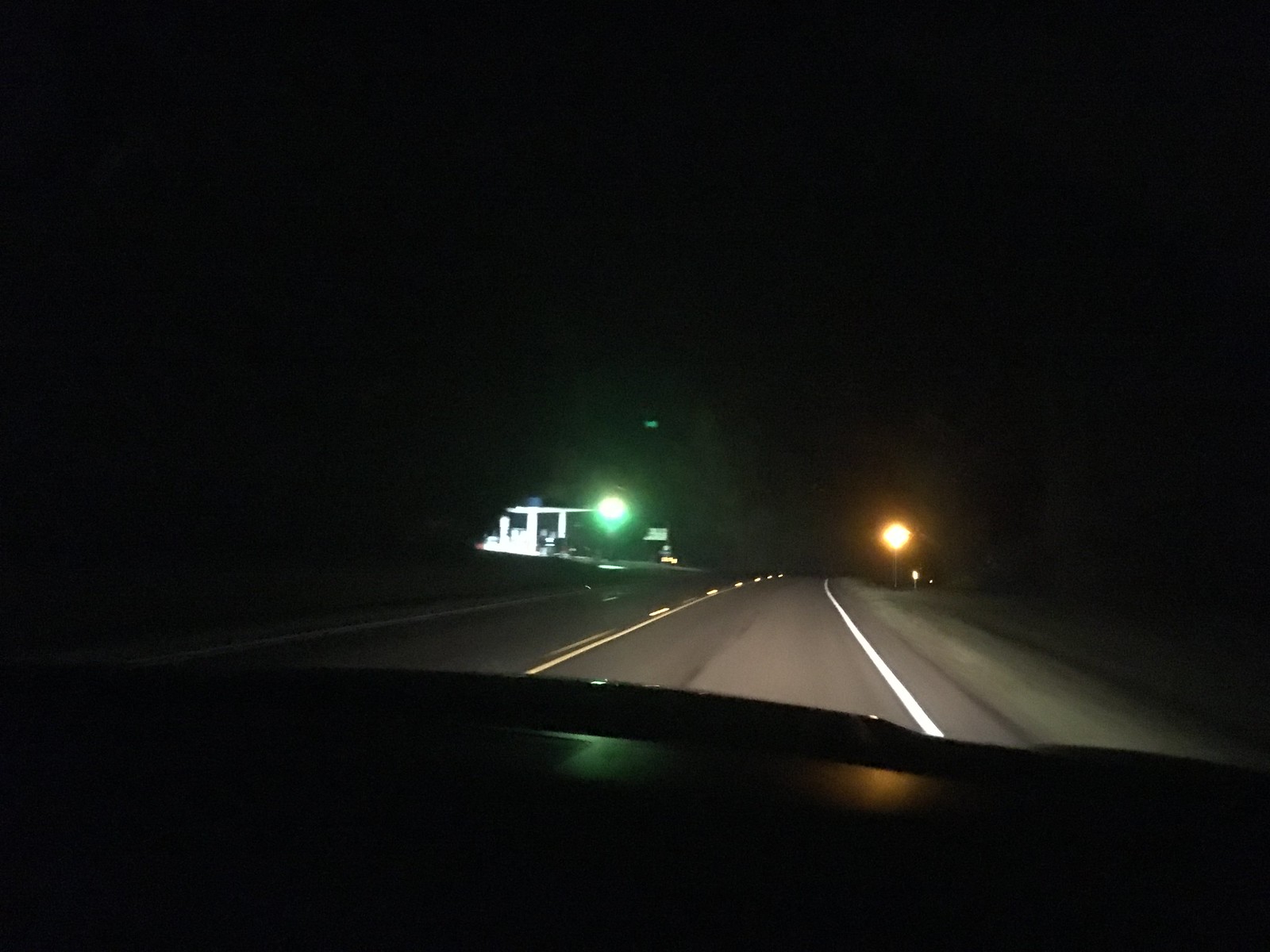A nighttime photograph captured from the passenger seat of a car through the front windshield features a desolate stretch of road ahead. On the right side of the road, a small white building—likely either a weigh station or a toll booth—stands illuminated. The road appears too narrow and isolated to support toll booths, leaning more towards it being a weigh station. A green light glows brightly in front of this building, casting a muted reflection on the pavement. On the opposite side of the road, a solitary yellow light adds a contrasting hue to the scene. The visibility extends only to the road, its shoulder, and the little structure; beyond these elements, the night’s darkness envelops everything, creating an atmosphere of tranquility and solitude.